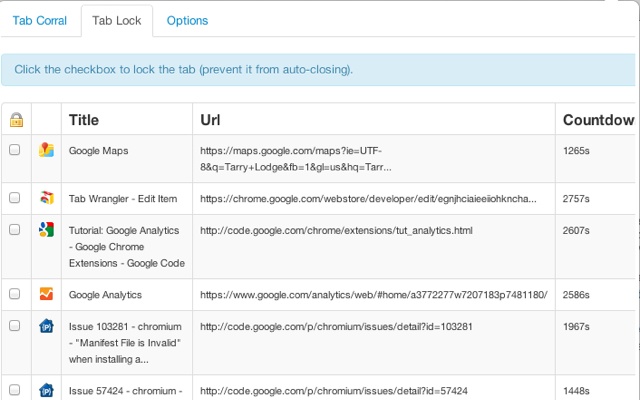The image depicts a website interface with a clean white background. At the top, there is a thin, fine line. Below the line, aligned to the left, it reads "TAB Corral" with "TAB" in uppercase letters starting with a capital 'T', and "Corral" starting with a capital 'C'. The "Tab Lock" option is highlighted.

Adjacent to "Tab Lock," the next option, "Options," is displayed in blue with a capital 'O'. The "Tab Lock" section extends downward, transitioning into a light blue banner that contains the following blue text: "Click the checkbox to lock the tab (Prevent it from auto-closing)."

Beneath the light blue banner, a chart is displayed. On the left side of the chart, there is an icon of a locked key. Each row below the locked key contains a checkbox that allows users to lock specific tabs. Adjacent to each checkbox, there is a graphic separated by a line. 

To the right, following the padlock, there are columns labeled "Title," "URL," and "Countdown." Each column is filled with corresponding entries, detailing the titles, URLs, and countdown times for the tabs listed.